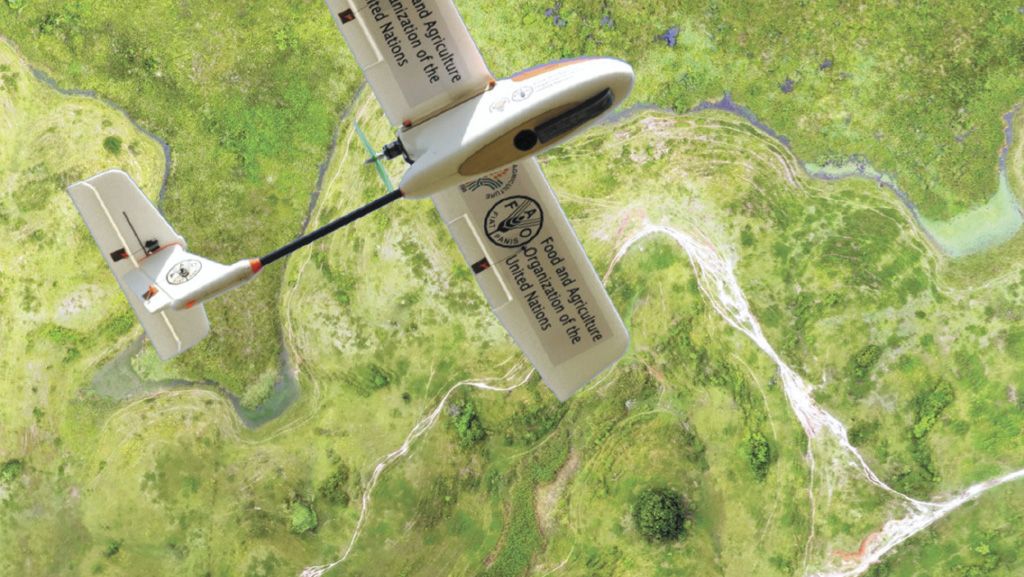This is a horizontally-oriented, top-down bird's-eye view photograph taken during the daytime. The centerpiece of the image is a small, white, and beige model airplane labeled with the "Food and Agriculture Organization of the United Nations" in dark blue font. This label is prominent on both wings of the model. The plane has a distinctive black rod connecting the tail to the fuselage, suggesting it's a scale model rather than a functioning aircraft. The background features a staged ground cover representing a vivid, green landscape that includes grass, trees, and prominent stream flows, evoking the appearance of rivers. The scenery is detailed and lush, embellished with some white areas on the grass, which might be pathways or design elements of the ground cover. The photograph is highly detailed, showing the intricate contrast between the meticulously modeled airplane and the vibrant, almost life-like landscape below.